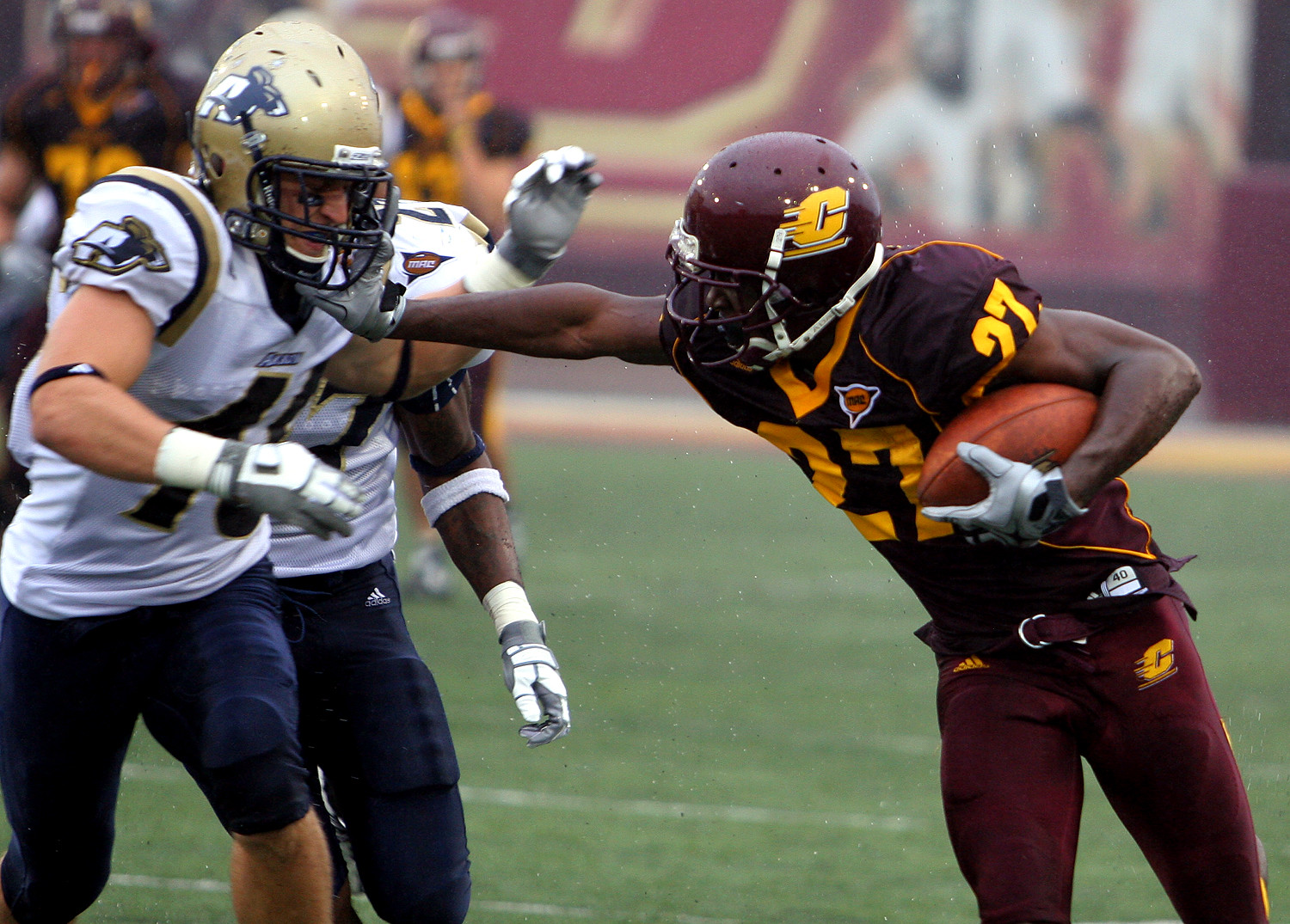This vibrant photograph captures an intense moment during an American football game, played on a lush green field under bright natural light. At the center of the action, a player from the team in deep maroon uniforms, accented with gold details and bearing yellow numbers along with a distinctive yellow "C" on their maroon helmets, is captured mid-play. This player tightly grips the football in his left hand while executing a powerful stiff arm against an opposing player. The opponent, donning a white jersey with gold accents, black pants, and a gold helmet, appears determined to tackle the ball carrier. Both teams sport Adidas gear, indicating the likely sponsorship. The blurred background reveals more athletes engaged in the game, surrounded by barriers and walls with red, yellow, and white logos, enhancing the scene's depth and intensity. The overall atmosphere is vivid and dynamic, perfectly encapsulating the competitive spirit of the game.